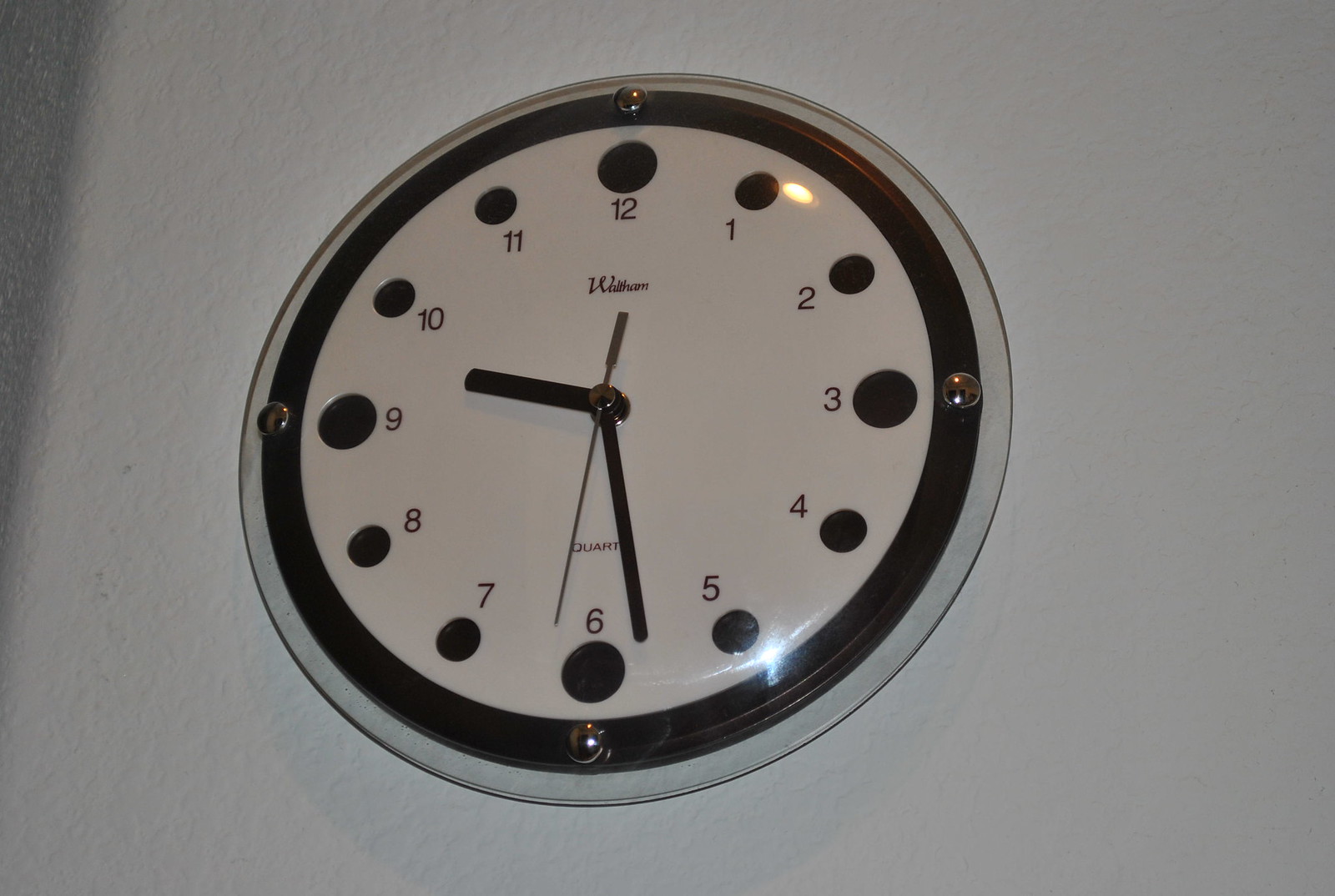A photograph showcases a round, flat clock mounted on a textured, painted white wall, with a light shining onto the clock's clear protective glass causing a noticeable glare. The clock itself has a white face bordered first by a thin light gray edge, then further encircled by a slightly thicker black trim. The clock is secured to the wall with four metallic studs or screws, placed at the 12, 3, 6, and 9 o'clock positions. Each hour is marked by bold black numbers, with smaller black dots above each number, and larger circular markers at the 3, 6, 9, and 12 positions. The clock features simple, straight black hour and minute hands, and a thin black seconds hand. Above the 12 o'clock position, the name "Watson" is inscribed in a small, partially cursive font, while "quartz" is written at the bottom above the 6 o'clock position. The clock's plastic construction and design give it an antiquated appearance.